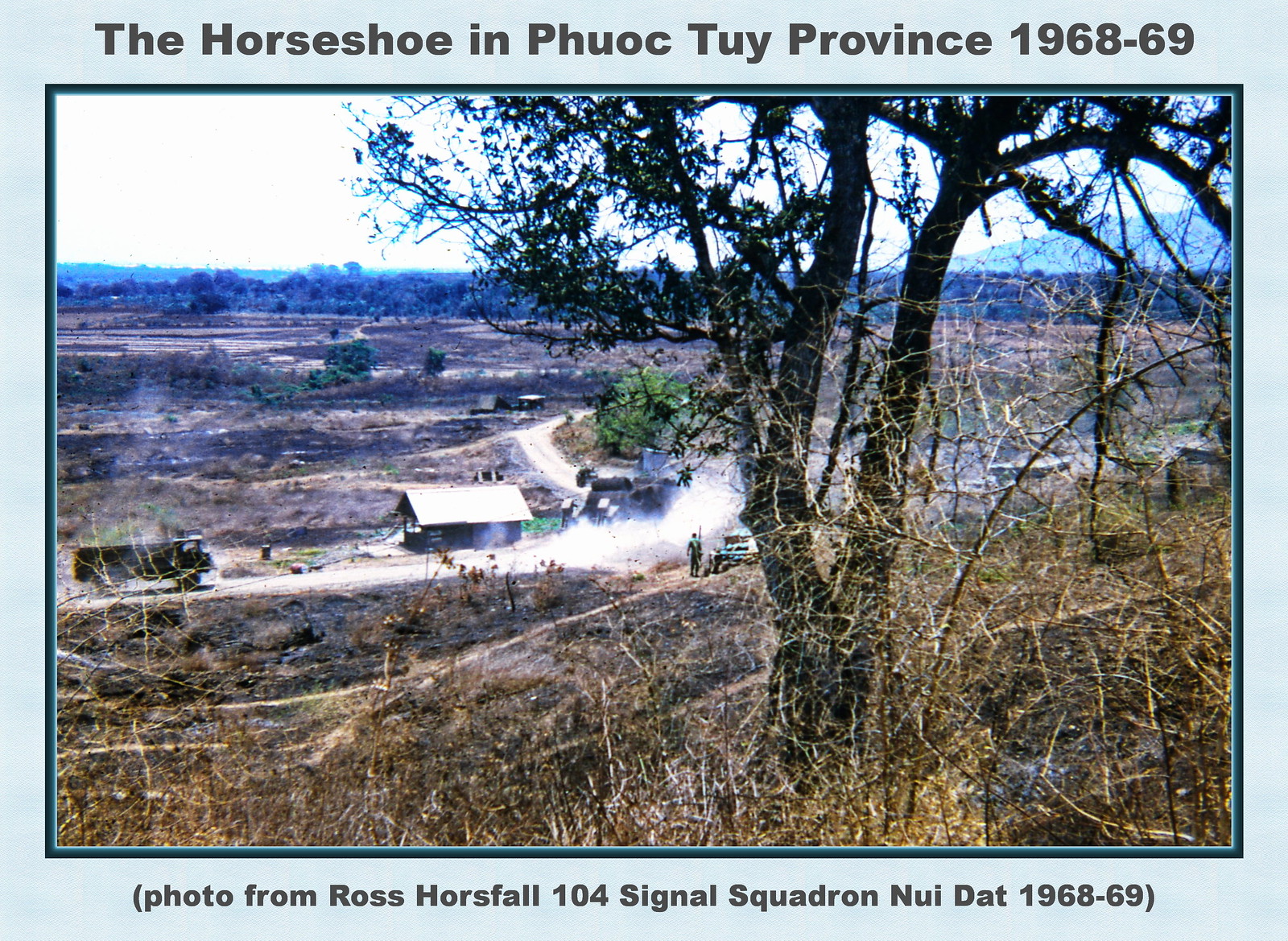**The Horseshoe in Phuoc-Tuy Province, 1968-69**

This detailed image portrays a rural village scene in Phuoc-Tuy Province during the years 1968-69. In the foreground, a tree stands prominently with many brown grasses blanketing the ground below it, both situated atop a hill. At the base of this hill near the center of the image, a house with a distinctive triangular white roof can be seen. To the left of the house, a black truck is parked. Further details emerge with the presence of a man, possibly armed, and an aqua-colored car to the right of the house, hinting at the context of the Vietnam War. The image is framed with a light blue border and an aqua matting beneath it, adding a layer of texture. The backdrop reveals a landscape filled with numerous trees and a range of mountains visible in the top right corner. The photograph is attributed to Ross Horsfall of the 104 Signal Squadron, Nguoi Dat, during the specified years.